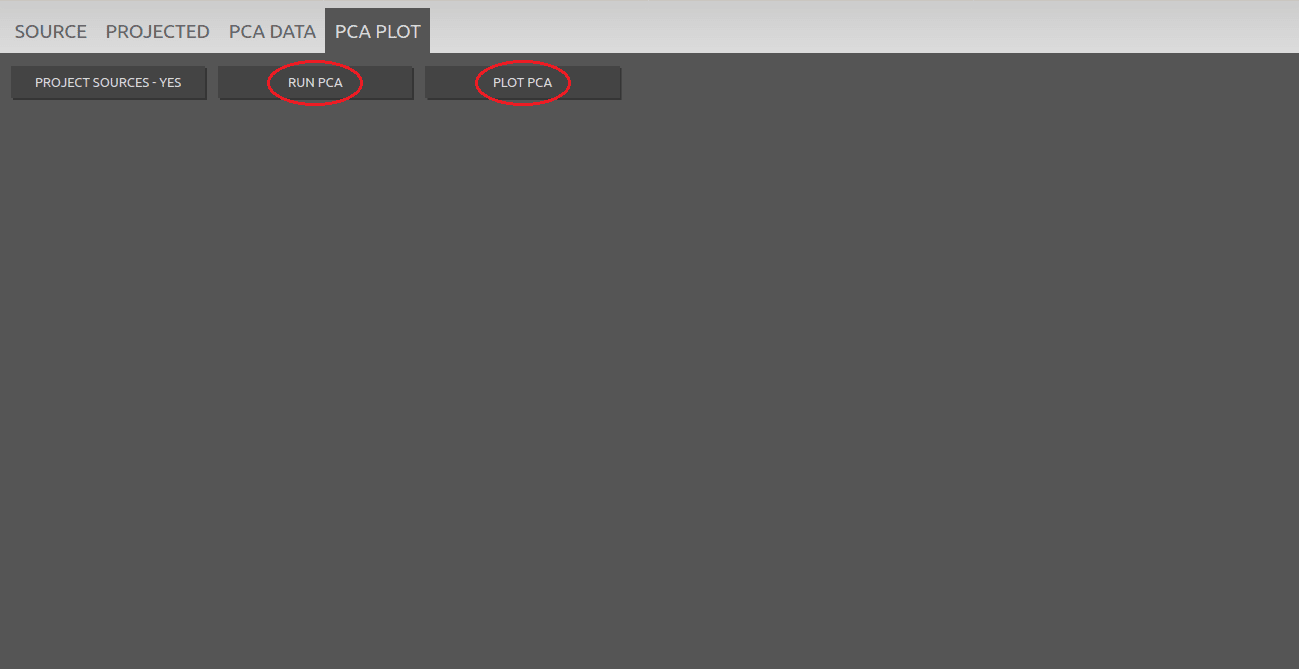The image features a predominantly dark gray background with a lighter gray section at the top, which contains four tabs labeled in all capital letters. From left to right, these tabs are labeled: "SOURCE," "PROJECTED," "PCADATA," and "PCAPLOT." The "PCAPLOT" tab is currently selected, which has changed its background to dark gray and its font to light gray.

Below the tabs, the main area is largely empty, which suggests that the screenshot might have been taken before any content was added or the work was completed. In this dark gray area, there are three dark gray rectangles, each with text in light gray or white font, also in all capital letters. The first rectangle reads "PROJECT SOURCES - YES". The second rectangle says "RUN PCA," while the third one is labeled "PLOT PCA." 

Interestingly, the last two rectangles ("RUN PCA" and "PLOT PCA") are each enclosed by red-outlined ovals, possibly indicating emphasis or importance. However, the reason for this highlighting is not provided, leaving it unclear whether the ovals were drawn by the person annotating the image or were originally part of the interface design.